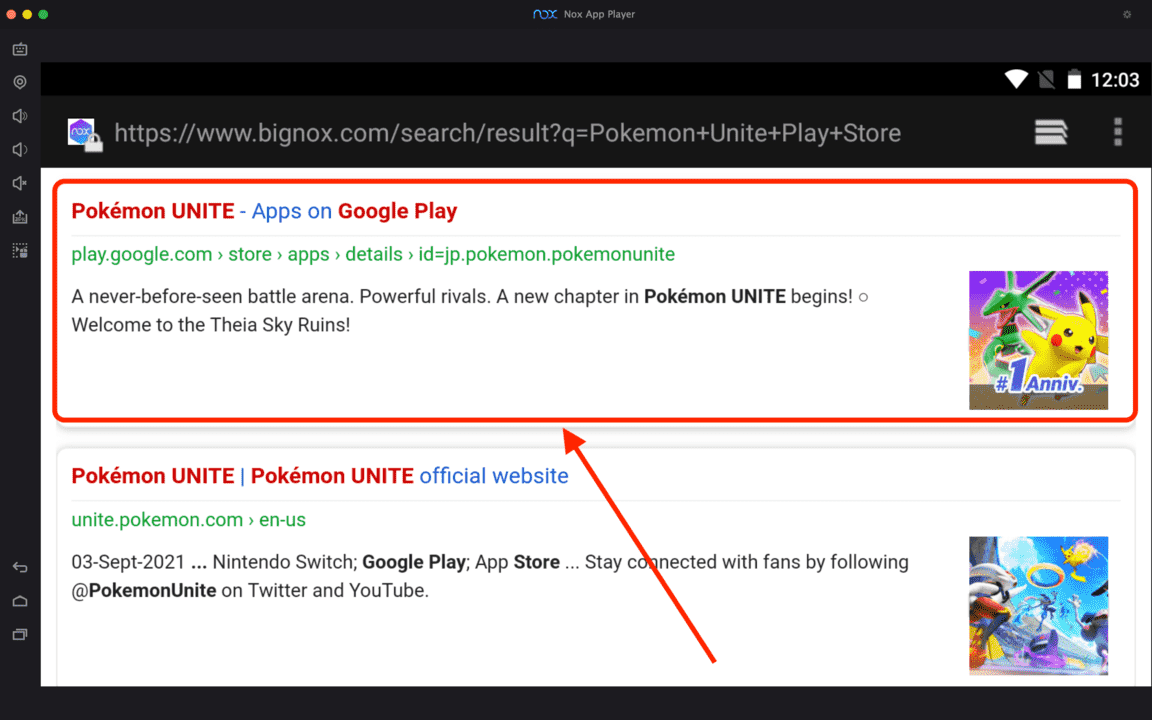Screenshot of a web page primarily displaying two listings related to Pokémon Unite.

**Background and General Layout**:
- The background of the web page is black, which contrasts with a prominent white box in the foreground containing the listings.
  
**Top Listing**:
- **Highlighting**: The top listing is circled in red with a red arrow pointing towards it.
- **Title**: The title reads "Pokémon Unite" in red font, immediately followed by "Apps On" in blue font, and concludes with "Google Play" in red font.
- **Link**: Below the title, there is a green link: "play.google.com > Store > Apps > Details > ID=JP.Pokemon.PokemonUnite".
- **Description**: The description text is in black and states: "A never before seen battle arena, powerful rivals, a new chapter in Pokémon Unite begins. Welcome to the Theia Sky Ruins."
- **Image**: To the right of this text, there is a cartoon-like square image featuring two Pokémon set against a multicolored background. The text in front of the creatures reads "1 ANNIV."

**Bottom Listing**:
- **Title**: The title again features "Pokémon Unite" followed by "Pokémon Unite official website".
- **Link**: Below the title is a green link: "Unite.Pokemon.com > EN-US".
- **Description**: In black text, the description reads: "03 September 2021... Nintendo Switch; Google Play; App Store... stay connected with fans by following @PokemonUnite on Twitter and YouTube."
- **Image**: To the right of this listing, there is a smaller square image. Although the details are indistinct, it appears to depict a colorful Pokémon battle scene.

**Header and Navigation**:
- **URL**: Above the white box, the URL displayed is "HTTPS://www.bignox.com/search/result?Q=Pokemon+Unite+Play+Store".
- **Icons**: On the left side of the header, there are small icons. Additional icons are present on the right, likely for menu options.
- **Status Indicators**: Above these icons, there are indicators for battery, signal strength, and the time (12:03).